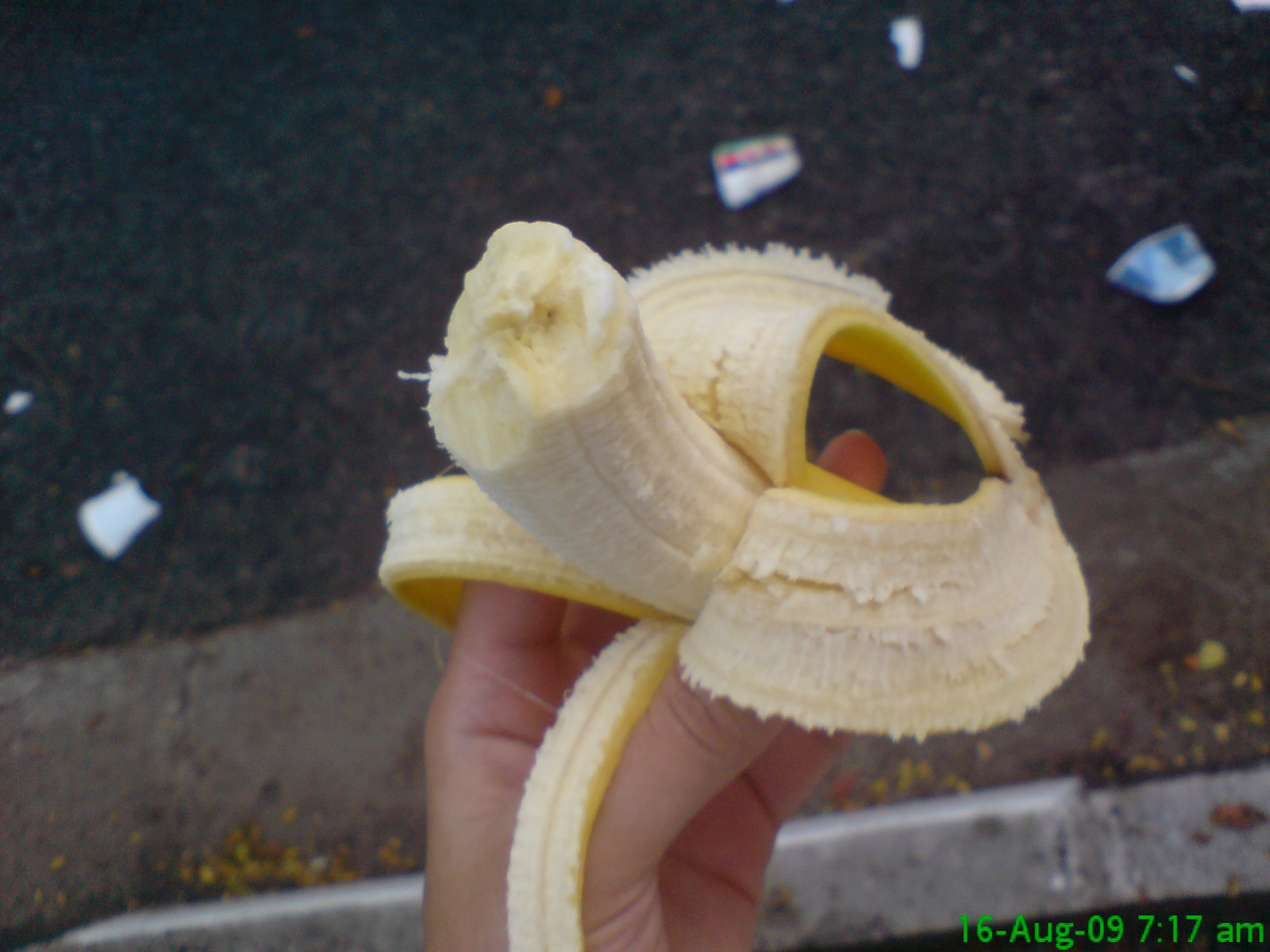This grainy photograph, dated 16-AUG-09 at 7:17 a.m., captures a close-up of a person's hand with light-colored skin holding a partially eaten banana. The inside of the banana peel reveals a fuzzy texture, as does the half-eaten banana itself. Below the hand, a street is visible, scattered with various debris, including yellow and orange leaves. Notably, there are two cups: one with a white base adorned with orange, blue, and green details, and another with a light blue body featuring dark blue accents. The pavement shows visible cracking, adding to the scene's worn aesthetic.